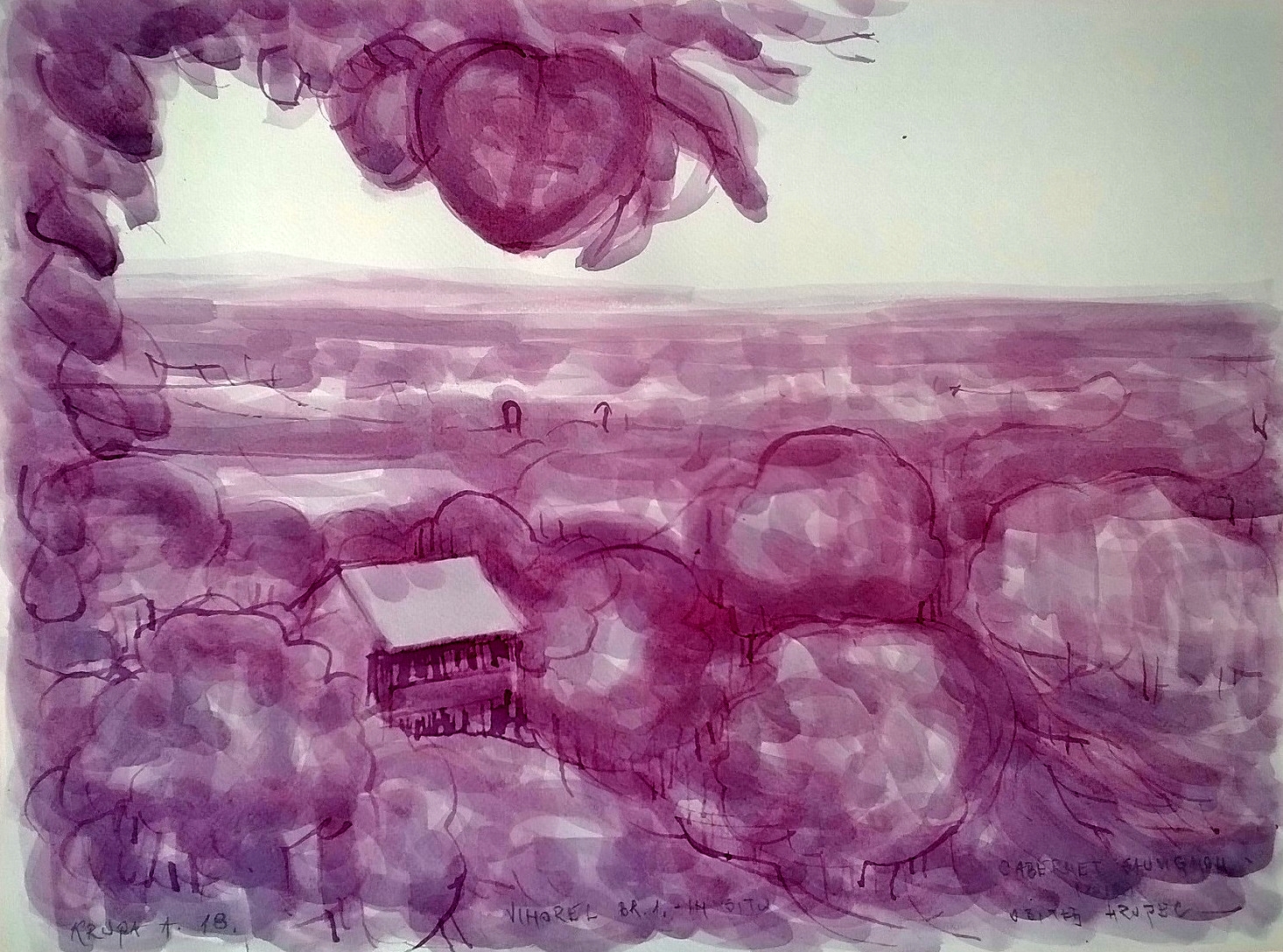The image depicts a distinctive and colorful painting, likely created with watercolor or oil-based paints, illustrating a serene country scene bathed in purple hues. Central to the composition, towards the bottom left of the canvas, stands what appears to be a country house, surrounded by various trees. The entire painting is suffused with shades of purple, pink, white, gray, and tan, imbuing the scene with a surreal and ethereal quality. Circles of purple designs are scattered throughout, adding to the abstract nature of the piece. In the background, the sky occupies the top fourth of the image, displaying a light blue hue with subtle hints of white, and is framed by distant mountains on the horizon. Notably, a fruit tree with visible fruit spans the upper portion of the painting. There is also some text, presumed to be the artist's signature, located at the bottom right, although it's difficult to read. This hand-painted artwork captures an outdoor setting under a clear, daylight sky.